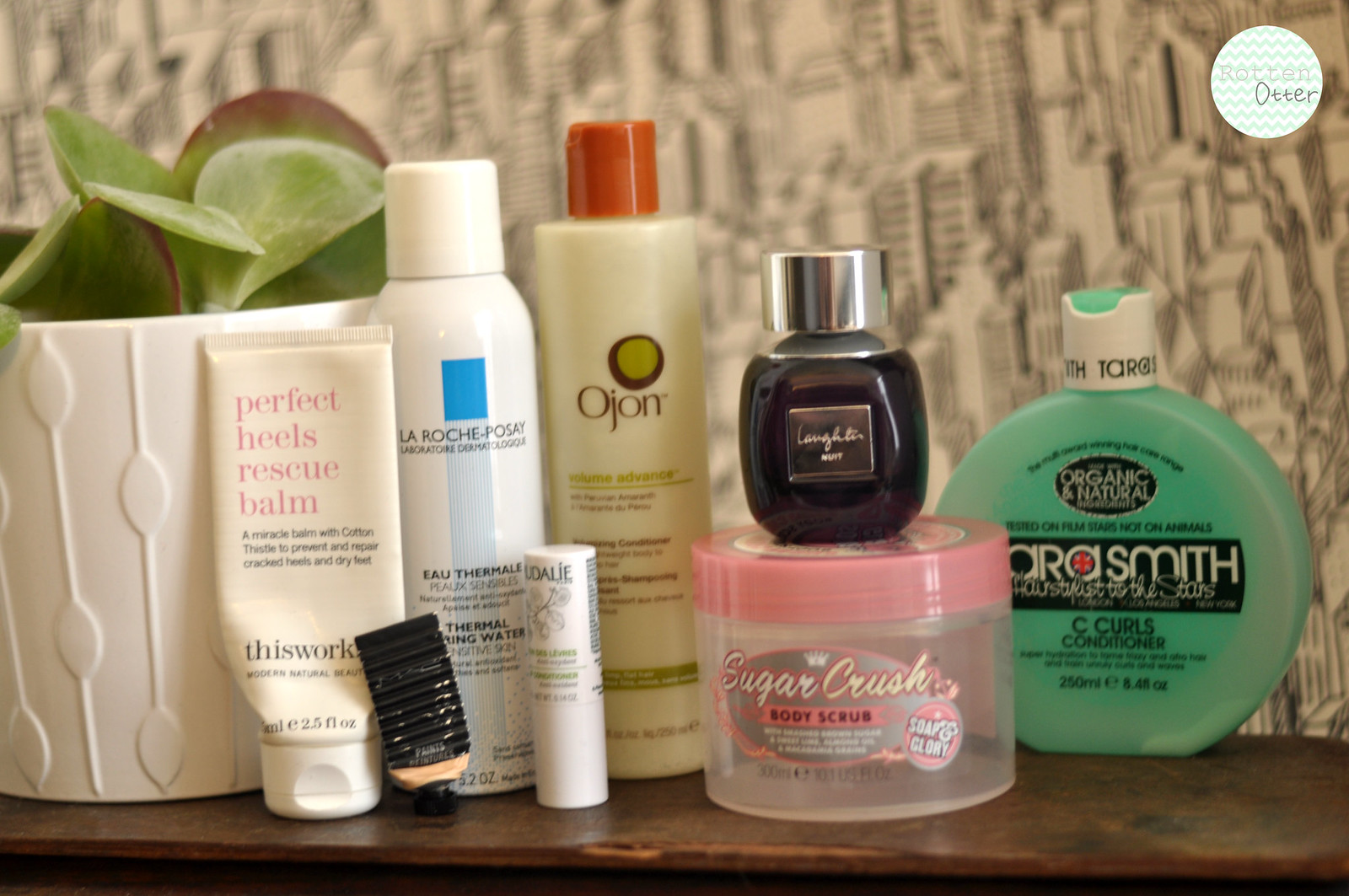On top of a dark wooden shelf, various hair and body products are neatly arranged against a backdrop of black and white illustrated cityscape wallpaper. From left to right, the first item is a tube of Perfect Heels Rescue Balm by This Works, a miracle balm with cotton thistle for preventing and repairing cracked heels and dry feet. Next is a bottle of La Roche-Posay Thermal Spring Water spray. To its right stands a bottle of Ojon Volume Advance volumizing conditioner. Further along, a small bottle of Laughter Nuit, which could be either perfume or body oil, is stacked atop an empty container of Soap & Glory Sugar Crush body scrub. The final item on the right is a distinctive round mint green bottle of Cara Smith Sea Curls Conditioner, labeled as organic and natural.